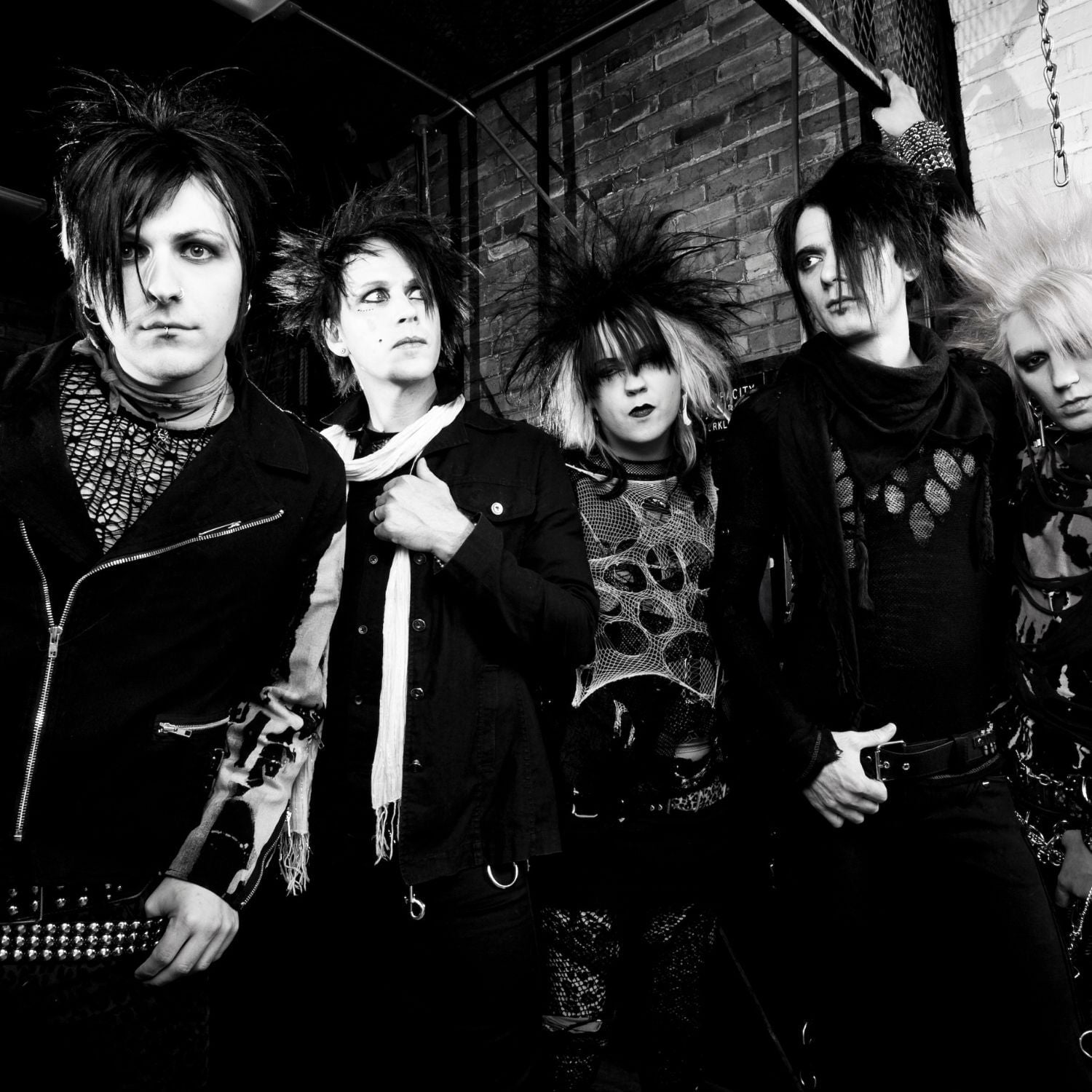This black and white photograph likely serves as a promotional image for a band with an emo or gothic aesthetic. Set against the backdrop of a brick wall, the image is infused with darkness and shadows, enhancing the moody, monochromatic theme. A chain dangles from the ceiling on the right side, adding to the edgy atmosphere. 

The band comprises five members, each sporting distinctive, heavily waxed, spiky hair that often covers one or both eyes. Starting from the left, the first member wears a black zipped hoodie over a netted shirt, accentuated by a spiked belt, with their left hand resting in the belt. Next to them is a person with black spiky hair and a white scarf, paired with a black jacket and pants. The central figure features striking black and blonde two-tone spiky hair, sporting a fishnet top and black pants.

To the right of the central member, another individual wears a black long-sleeve shirt with a mesh cutout in the middle. This member also has longer black hair. The last person, partially out of the frame on the far right, appears to be a woman with a near-mohawk of blonde hair. Some of the members have pierced lips, and all are dressed predominantly in black, solidifying their gothic and emo appearance.